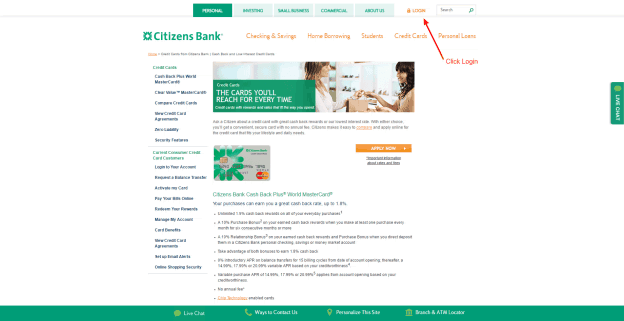This image displays a promotional webpage for Citizens Bank. At the center, there's an attention-grabbing arrow pointing towards the "Login" button, indicating the option for users to log into their accounts. The highlighted services include checking and savings accounts, home borrowing options, student financial services, credit cards, and personal loans.

In the foreground, two women appear to be exchanging an item, symbolizing customer service or transaction. The tagline “The cards you will reach for every time” suggests a focus on credit card offerings. Due to the low quality of the image, some text remains illegible, making certain details unclear.

At the bottom of the webpage, there's a prompt for a live chat feature with the inviting phrases “Please do contact us” and “Personalize the site,” encouraging user engagement and personalized banking experience.